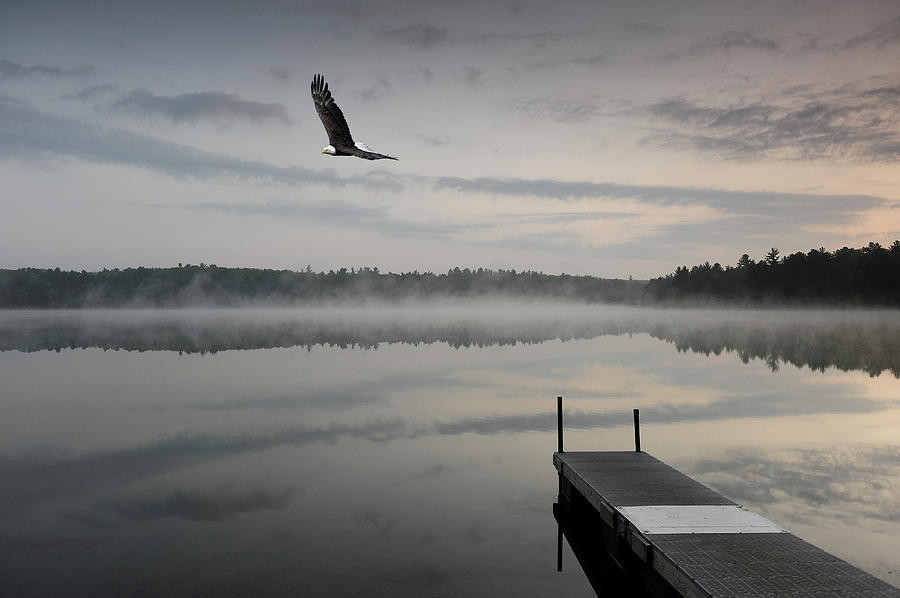This photograph captures a serene and misty morning over a tranquil lake, enveloped in drab and dreary hues of gray, charcoal, and brown that lend an almost monotone quality to the scene. A wooden deck extends from the bottom right-hand corner into the lake, with a noticeable patch where white boards replace the original brown ones, drawing the eye. Mist rises gently off the lake, adding a sense of ethereal calm to the landscape. Across the water, the distant tree line, likely composed of towering pines, stretches to the horizon, their silhouettes dark against the soft light of early morning. Above this tranquil setting, a majestic bald eagle with distinct white head wheeling gracefully through the sky, positioned in the top left third of the image, accentuates the wilderness of the scene. The overcast sky, covered with patches of clouds that cast subtle shadows, reflects dimly in the still, calm waters below, emphasizing the peaceful and undisturbed beauty of nature.